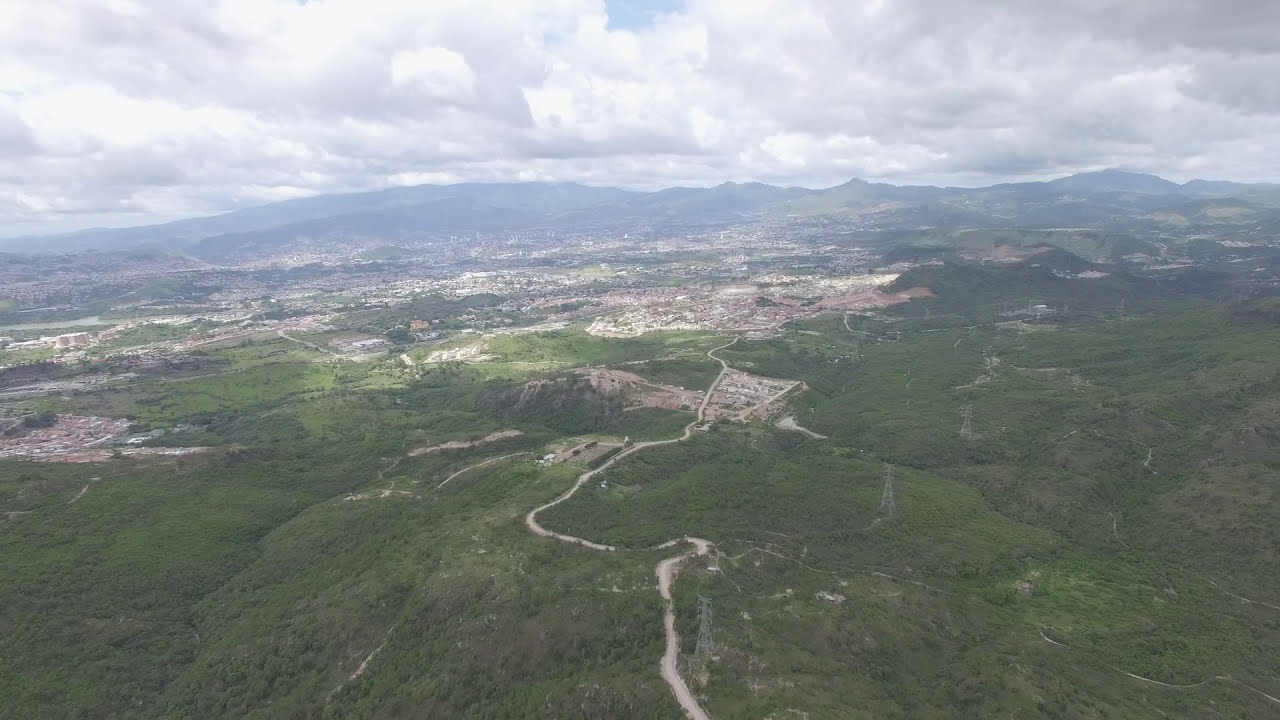This aerial photograph captures a lush, green valley nestled beneath a towering mountain range. At the top of the image, densely packed white and gray clouds dominate the sky, casting a hazy shadow over the landscape below. The mountain range, stretching from left to right, becomes increasingly rocky towards the right. Below, the scene transitions from rocky, dark gray, and blue hills to a sprawling valley dotted with tiny, light tan homes that blur together, indicating a town or small city. Winding roads traverse the valley, interspersing the green foliage and rolling hills. One prominent road zigzags from the lower center of the image, connecting the verdant hills to the distant urban area. The image beautifully contrasts the untouched green expanses with pockets of human habitation, all viewed from an airplane-like perspective high above.